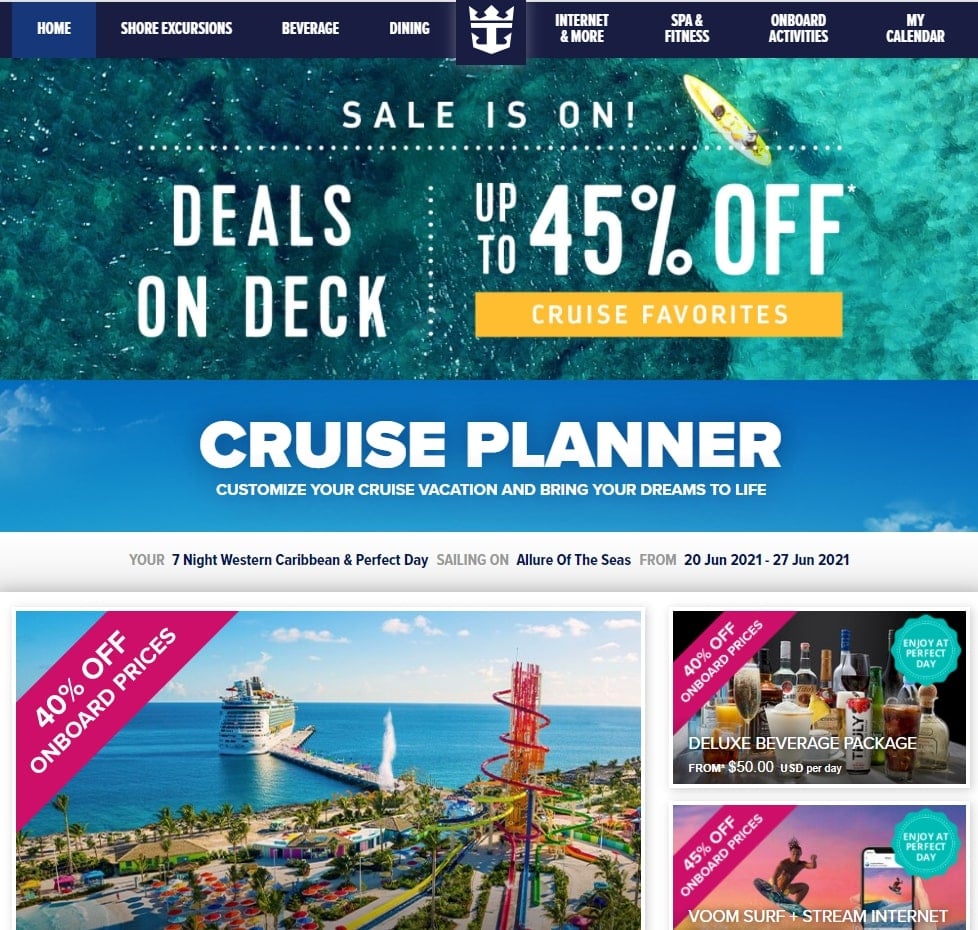The homepage of this travel website features a user-friendly cruise planner designed for organizing your vacation. The top of the page has a dark blue banner with navigation tabs including Home, Shore Excursions, Beverages, Dining, Internet, Spas and Fitness, Onboard Activities, My Calendar, and a distinctive anchor with a crown icon.

The Home tab is highlighted in light blue, indicating the current section. Below this banner, a vibrant image of a turquoise kayak on water is prominently displayed. The image has a mixture of light and dark water hues, overlaid with white text announcing "The Sail is On: Deals on Deck, Up to 45% Off." Beneath the text, an orange button labeled "Cruise Favorites" invites users to explore popular options.

Further down, another banner depicts a bright blue sky with white text proclaiming, "Cruise Planner: Customize Your Cruise Vacation and Bring Your Dreams to Life." Below this, detailed information about an upcoming cruise is provided: "Your Seven Night Western Caribbean and Perfect Day Sailing on Allure of the Seas from 20 June 2021 through 27 June 2021."

At the bottom of the section, there is an image that seems to resemble an amusement park, possibly indicating additional activities or destinations available on the cruise.